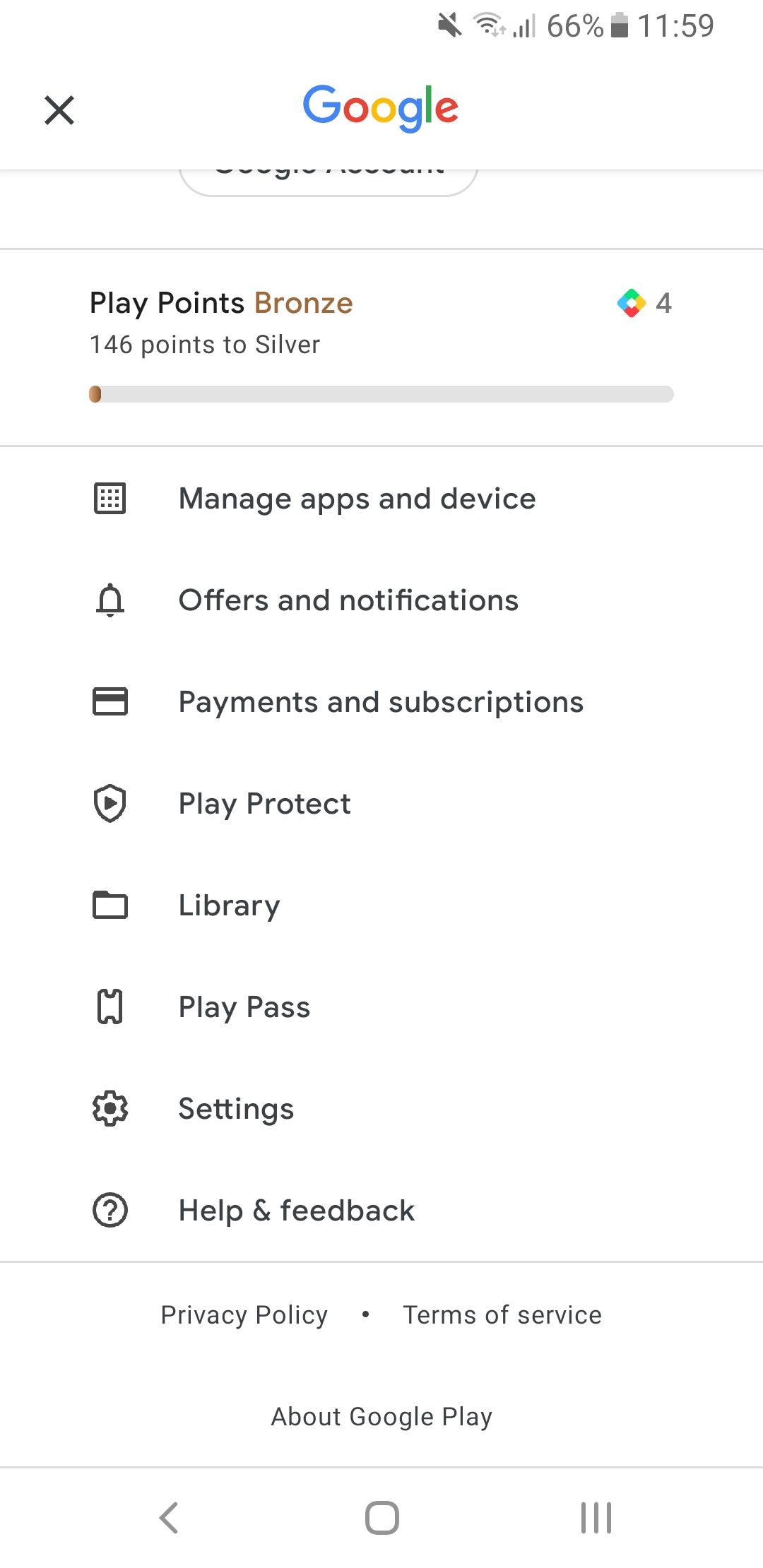The image showcases someone's Google settings on their phone, with a user interface centered around the Google Play app. At the top of the screen, the word "Google" is prominently displayed in the center. Directly below, the screen shows the user's Play Points status, indicating "Play Points Bronze" and noting that 146 points are needed to reach Silver status.

The interface is organized with various icons and labels in a list format. The first line has a gear icon labeled "Manage apps & device". Following this is a line with a bell icon next to the text "Offers and notifications". 

Next, there is a credit card icon along with the label "Payment & subscriptions". Further down, a shield icon with a play button in the center is associated with "Play Protect". Below this, a folder icon is labeled "Library".

The next icon is shaped like a cinema ticket and labeled "Play Pass". Following that is a settings wheel icon labeled "Settings". Finally, a question mark within a circle, labeled "Help & feedback", concludes the list of icons.

At the bottom of the page, there are links for "Privacy Policy", "Terms of Service", and "About Google Play". Additionally, navigation icons include a left-facing arrow, an unspecified circular icon, and a three-bar menu icon.

This appears to be the settings and management interface for the Google Play app on the user's phone, detailing various account and app management options.